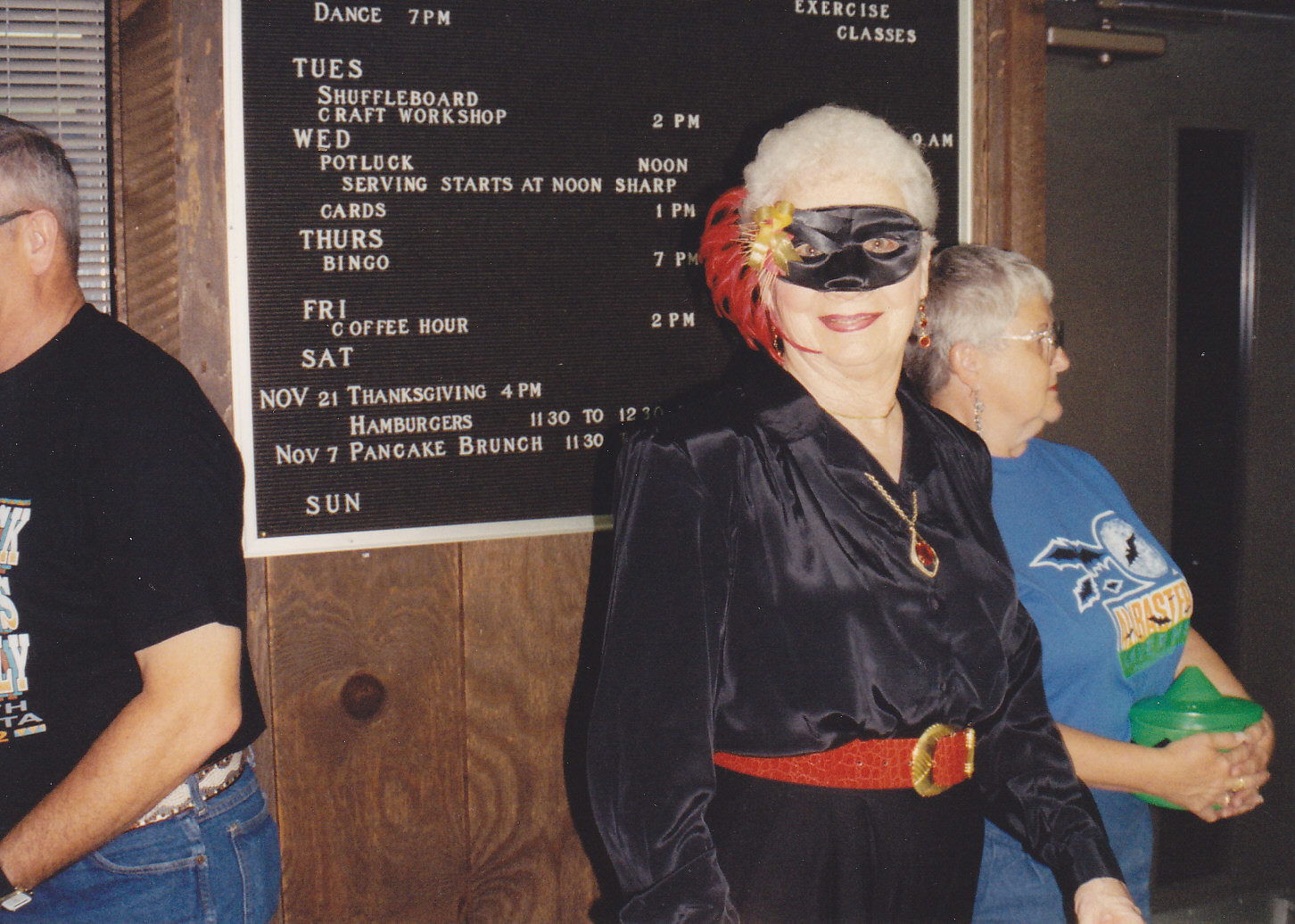In this wide rectangular image, a group of people is gathered in front of a black event schedule posted on a vertically planked wooden wall. The man on the far left, who is partially out of the frame, is wearing blue jeans and a black shirt and is facing left. A window with white blinds is visible near him in the top left corner. In the center, an older woman dressed in festive attire, likely for a Halloween or costume party, gazes directly at the camera. She has short silver hair and wears a black masquerade mask adorned with red feathers. Her outfit includes a black silky blouse, a red belt with a gold buckle, black pants, and red dangly earrings. She also sports a gold necklace with a pendant featuring a red gem.

To her right, a shorter woman stands, wearing a light blue shirt with a graphic of bats over a moon. She has short gray hair, glasses, and silver earrings, and is holding a plastic container. The event board behind them lists various activities such as shuffleboard, craft workshops, potlucks, bingo, and coffee hour, with specific dates and times, including significant events like "Thanksgiving, 4 p.m., November 21st."

The setting appears to be indoors, in a dimly lit room, giving the image an old photo feel. The variety of colors in the image includes tan, brown, black, red, gold, blue, green, and yellow.